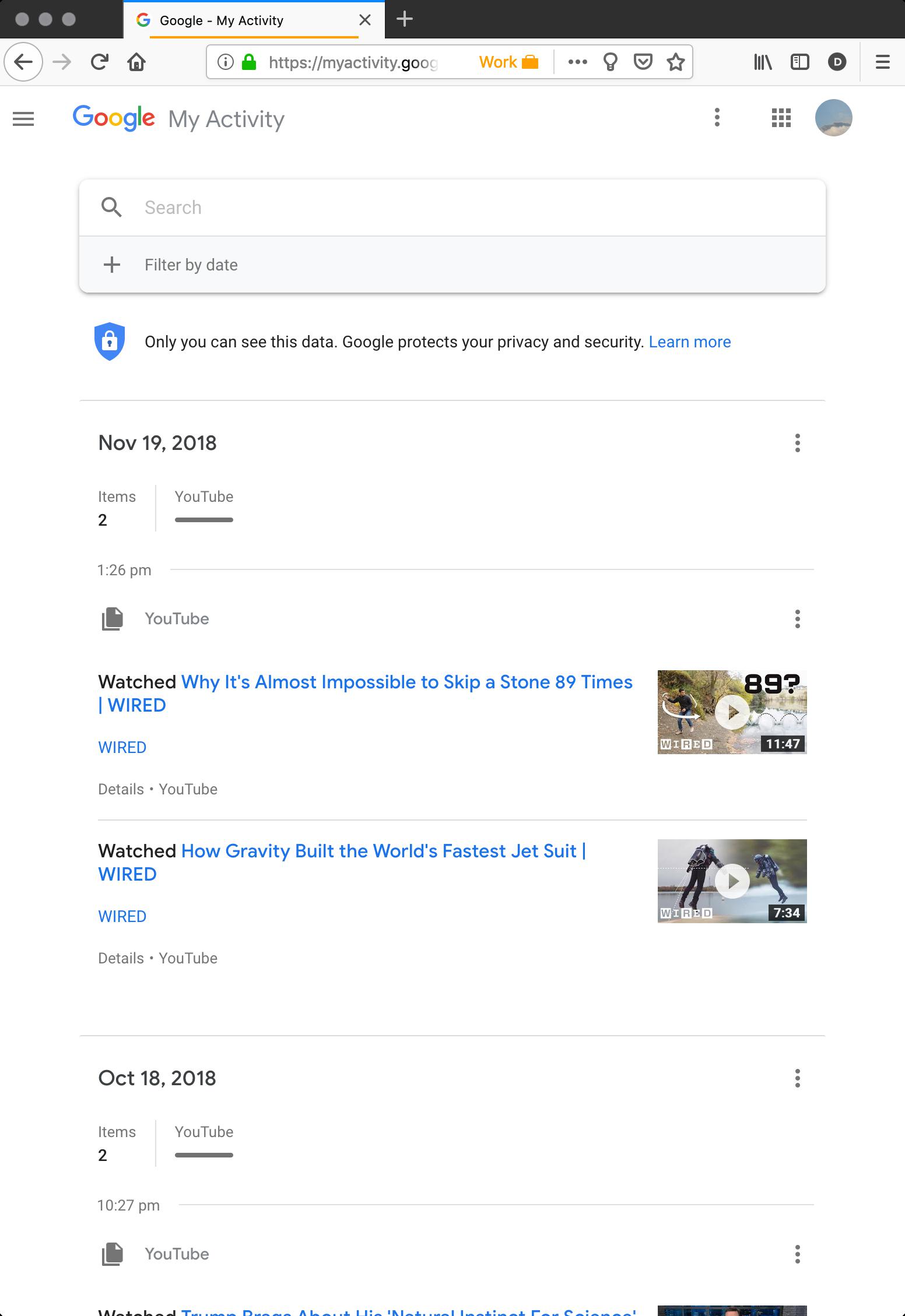Screenshot of Google MyActivity Page

This image captures a Google MyActivity page detailing user activity on a white background with blue and black text, along with thumbnail images from viewed videos. At the top, a black bar features three gray dots on the left. Adjacent is a blue bar that reads "Google - MyActivity."

Below this bar is a toolbar containing a refresh icon, a home icon, a search bar, and additional icons. The next section presents the Google logo in vibrant colors next to the text "MyActivity." On the right are three vertical dots, the nine-circle Google Apps icon, and a profile picture.

Underneath, there's a search bar with a magnifying glass icon, followed by a gray bar with options such as a plus sign and "Filter by date." The activity log starts with the date November 19, 2018, listing two items under YouTube:

1. At 1:26 PM, the video titled "Why It's Almost Impossible to Skip a Stone 89 Times" from Wired. The thumbnail shows a man throwing a stone with the number "89?" overlaid.
2. The second video, "How Gravity Built the World's Fastest Jet Suit" from Wired, shows two individuals wearing dark clothing and jet packs. The video length is 7:34.

The next date in the log is October 18, 2018. It lists activities from YouTube, beginning with one entry at 10:27 PM. The remainder of this date’s details are not visible in the screenshot.